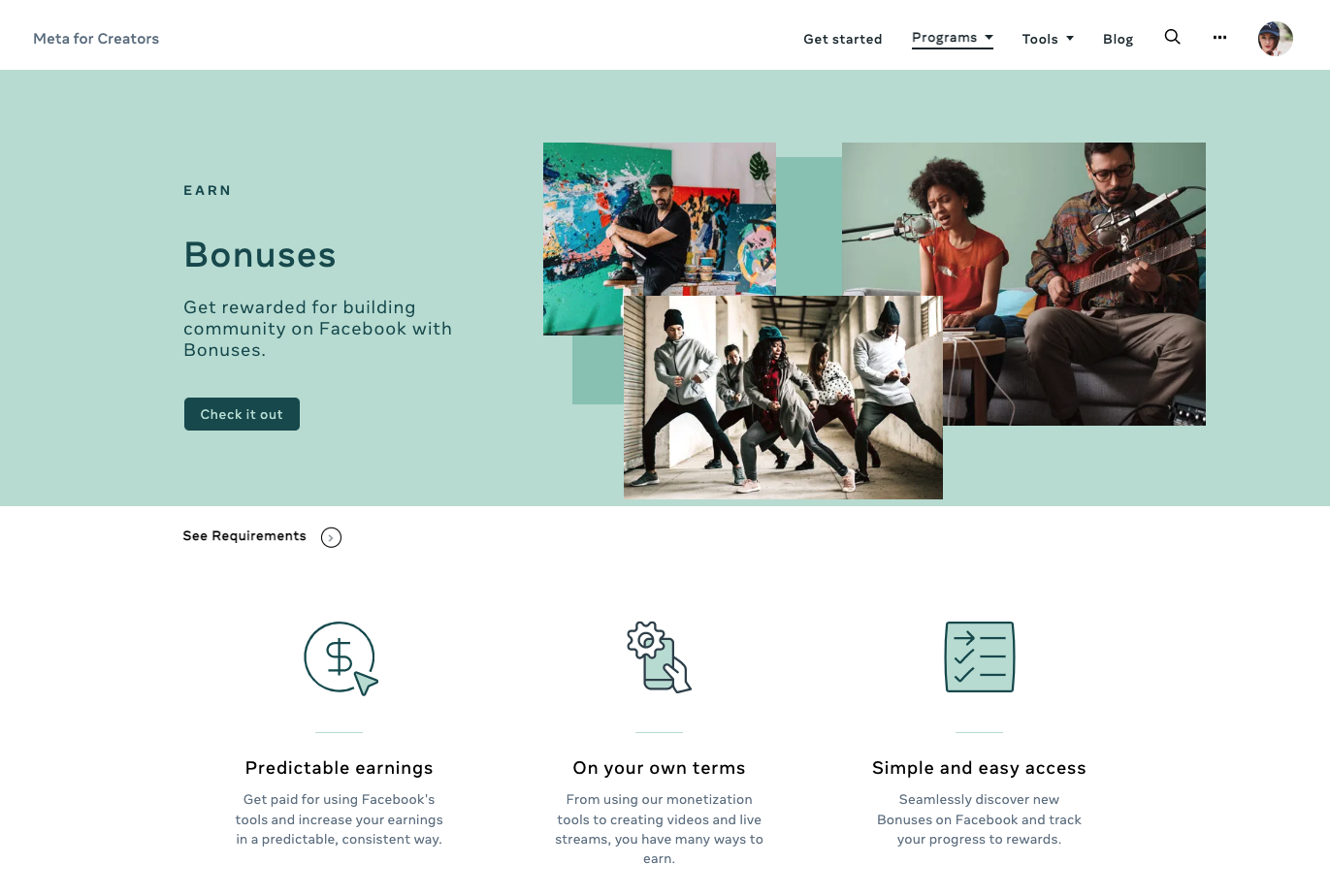Here is the cleaned-up and detailed caption for the image:

---

A website screenshot showcasing the "Meta for Creators" platform. At the top left corner, it displays "Meta for Creators," while the top right features a "Get Started" button. The navigation bar includes options: "Programs" (selected), "Tools," "Blog," and a magnifying glass for search. Below the navigation bar, a prominent mint green banner reads "Earn Bonuses" and encourages users to "Get rewarded for building community on Facebook with bonuses. Check it out."

To the right of the banner are three photographs: one depicts a fair-skinned man seated in front of several canvases he appears to have painted; another shows five people performing a dance; the third image features a dark-skinned woman playing a keyboard and singing alongside a light-skinned man playing a guitar. 

Below the banner is a white section detailing two main benefits. The first, "Predictable Earnings," highlights how creators can get paid for using Facebook's tools and consistently increase their income on their own terms. The second, "Simple and Easy Access," emphasizes the seamless discovery of new bonuses on Facebook and the ability to track progress towards rewards. The overall layout is wider than it is tall, and there are no animals present in the image.